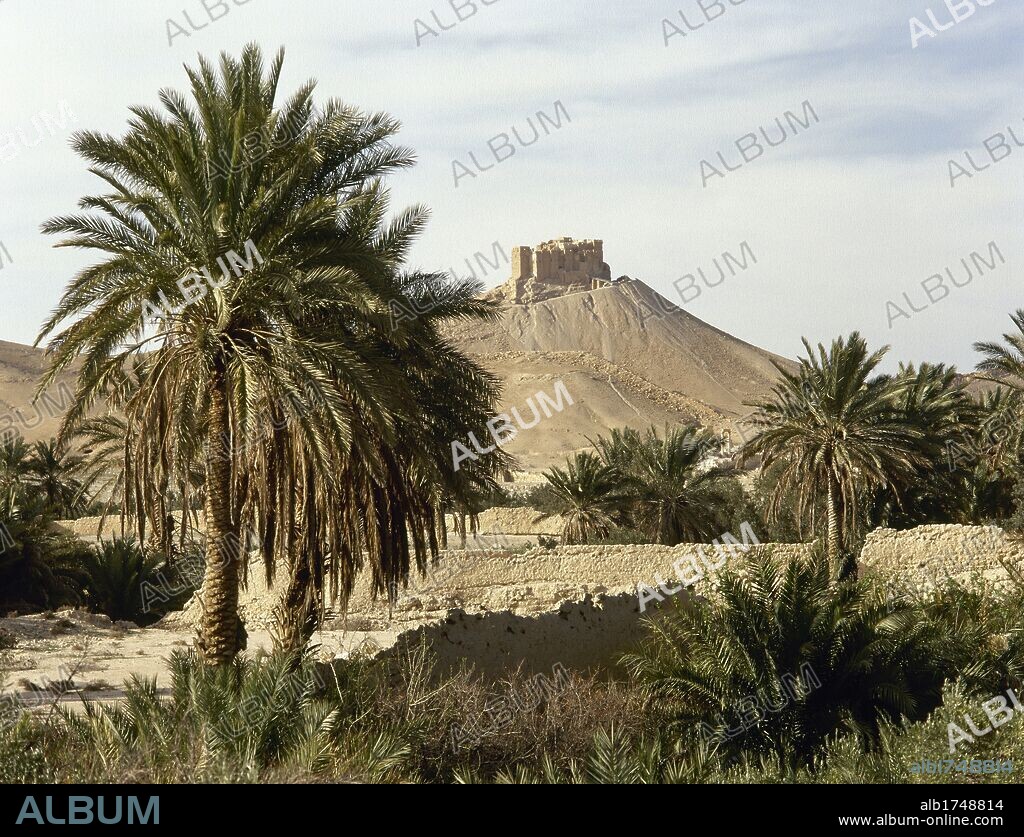The image is a digital photograph dominated by a desert scene with a dystopian atmosphere. In the foreground, there are several trees and bushes, typical of an oasis, characterized by a mix of green foliage amidst the tan and beige hues of the sand and desert. Above this vegetation, the sky appears hazy with white clouds. The middle and background of the photograph reveal an old, ruined structure, possibly a castle, situated atop a distant mountain or hill. This structure is shrouded in mystery, with no clear entrance visible. Watermarks labeled "ALBUM" are prominently slanted across the image. At the lower portion, a black stripe runs horizontally, with the word "ALBUM" in teal letters on the lower left corner, and "ALB1748814 www.album.online.com" in white font on the lower right corner. In the photograph itself, over the lower elements, the code "PIB1748814" is visible.